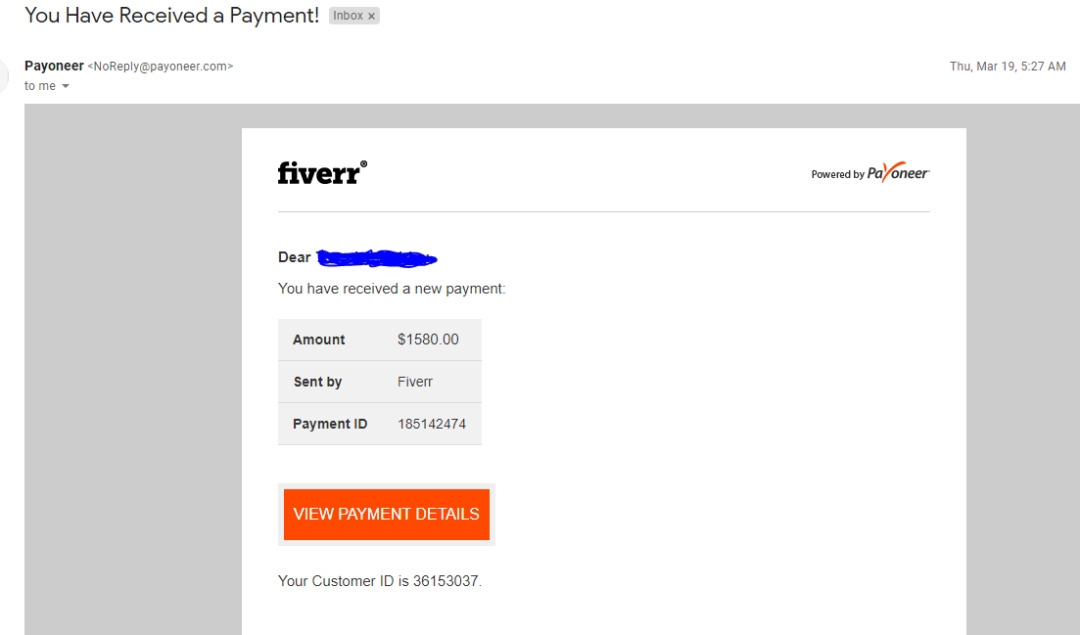This image is a screenshot of an email notification. At the top left, in bold black text, it reads "You have received the payment!" Adjacent to this message, on the right, there's a small, light grey rectangular tab labeled "Inbox" in slightly darker grey text, along with a little cross mark to close the tab.

Below this, partially visible on the far left edge, is a portion of a circular profile picture. To the right of this image, the sender's name "Payoneer" is displayed in bold black text. Underneath, the sender's email address, "noreply@payoneer.com," appears, followed by "To: Me." On the far right, the date and time "Thursday, March 19, at 5:27 AM" are noted.

In the main body of the email, the content showcases a notification from Fiverr, indicated in small caps as "FIVERR," highlighting information about a received payment. The email, powered by Payoneer and showing the Fiverr logo, states, "Dio," with the specific recipient's name obscured by a blue block. Below this, it declares, "You have received a new payment," amounting to $1,580, sent by Fiverr with the payment ID "1851-42474." 

Additionally, there's an orange tab below this message, inscribed in white with "View Payment Details." Finally, At the very bottom, another line provides, "Your Customer ID is 36153037."